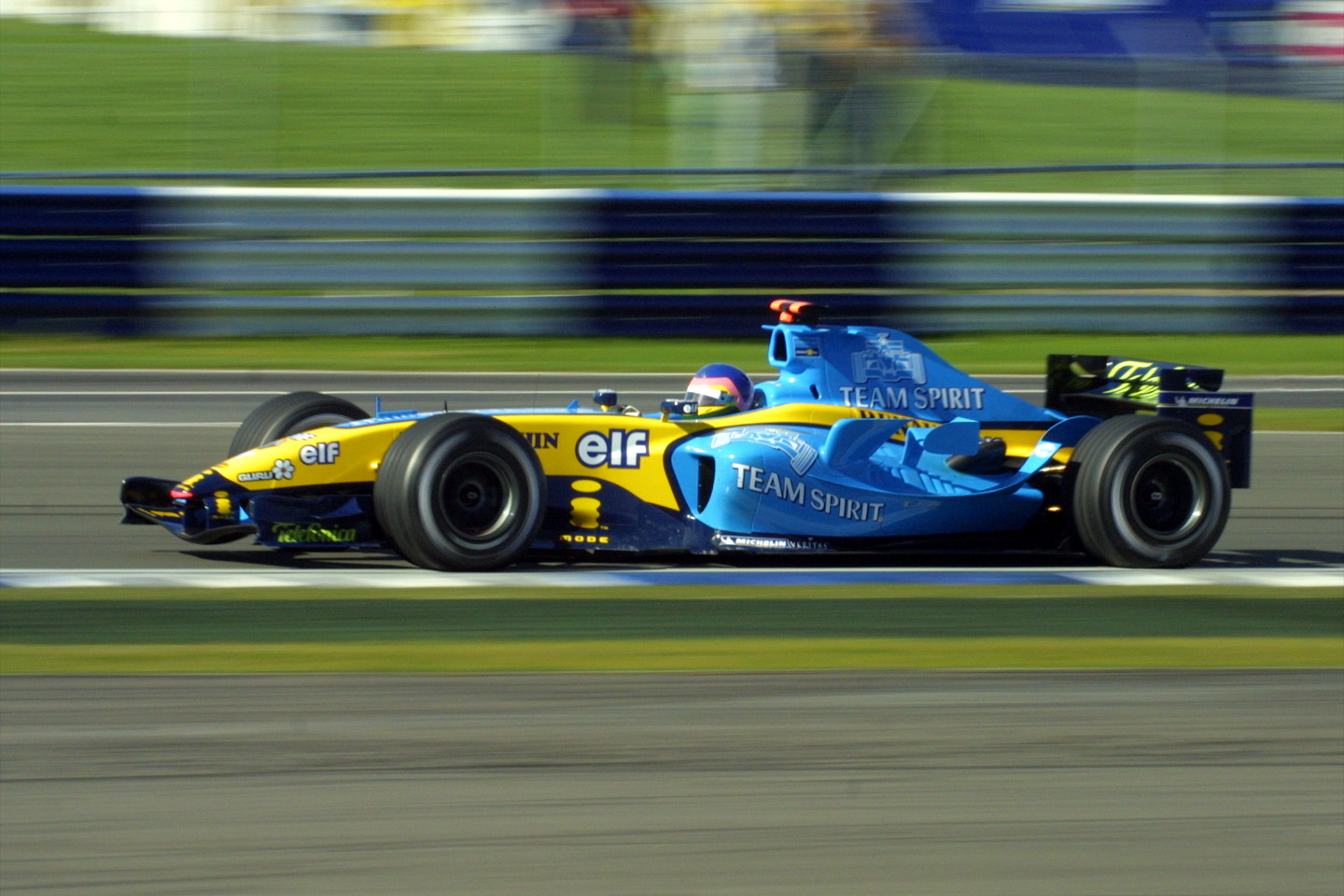A dynamic shot captures a race car speeding along a gray track, its blistering pace evidenced by the motion blur of its tires and the streaked background. The race car features a distinctive yellow front and a blue rear, adorned with numerous sponsor stickers, including prominent "ELF" branding in white. The rear also displays the words "Team Spirit" twice, in white lettering both at the top and bottom sections. A solitary driver, wearing a navy helmet accented with white, pink, and yellow, pilots the low-profile vehicle. Black tires hug the course closely, while a rear spoiler enhances its aerodynamic design. In the blurred background, green grass and a distant wall adorned with barely discernible signs further emphasize the car's high speed and the thrilling motion of the race.